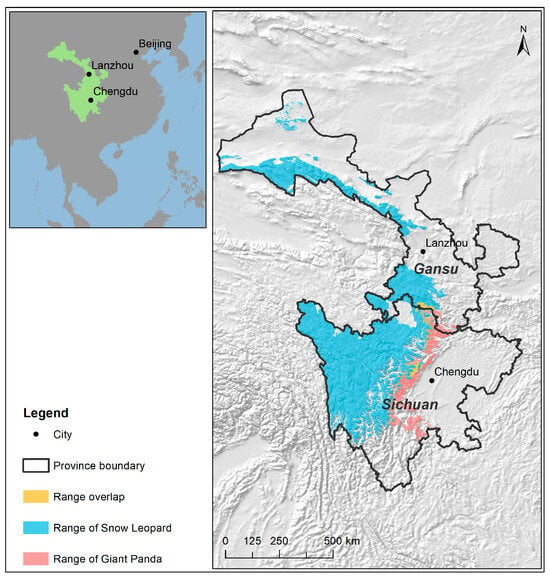The image is a detailed map layout with a thin black border. It consists of two primary sections: On the upper left, there's a smaller square featuring a zoomed-out map of China. Within this map, gray outlines show land and blue represents water, highlighting cities like Beijing, Lanzhou, and Chengdu with black text. Lanzhou and Chengdu are positioned in a bright green area. Below this section, a vertical rectangle contains a legend on a white background. The legend explains that a dot signifies a city, an open black rectangle denotes a province boundary, an orange rectangle indicates range overlap, a shaded blue area represents the range of snow leopards, and a shaded pink area signifies the range of giant pandas.

To the right, a larger vertical rectangle zooms in on this region, displaying a detailed gray-textured background with black outlines of provincial boundaries. This right section prominently shows Lanzhou in Gansu (G-A-N-S-U) at the top and Chengdu in Sichuan (S-I-C-H-U-A-N) at the bottom. Various shaded areas—blue for snow leopards, pink for giant pandas, and orange for their overlap—are clearly marked. Additional features include a compass symbol in the top right corner and a scale bar at the bottom, indicating distances up to 500 kilometers.